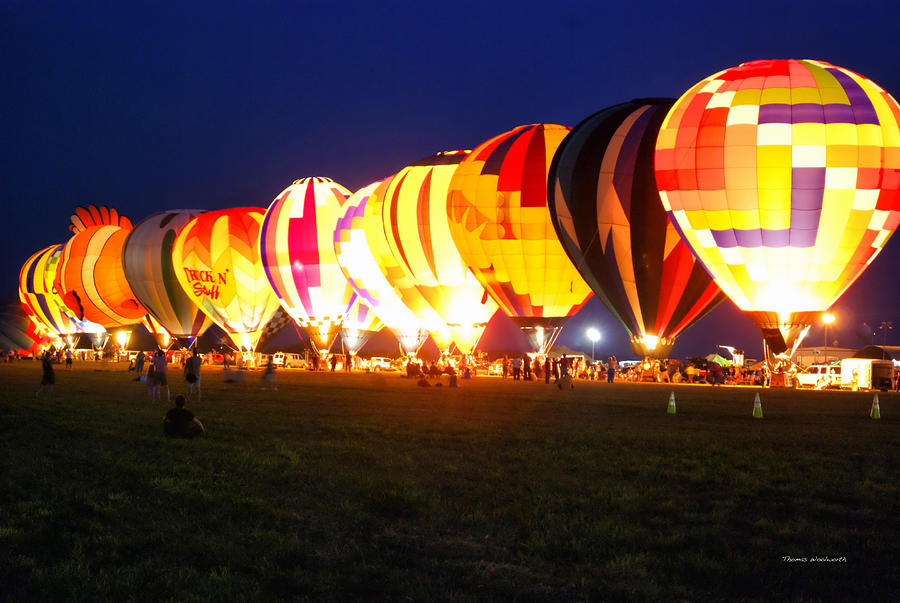This photograph, taken at pre-dawn, captures a mesmerizing scene of at least ten fully inflated, colorful hot air balloons aligned in a row on a flat field, with numerous vehicles and people milling around. The balloons are adorned with various vibrant patterns, including vertical stripes, checkerboards, Tetris-like colored blocks, and zigzag triangles, prominently featuring hues of yellow, orange, red, black, and white. One balloon intriguing stands out with a clownfish design, sporting orange, white, and black stripes and fins, while another appears to have a mohawk sticking out the top. Each balloon seems internally luminous, possibly due to the burning air heating elements at their bases, casting a warm glow in the early twilight. The scene is elegantly punctuated by small, white text in the bottom right corner of the image, where a signature of the photographer can be faintly discerned. The sky in the background hints at the approaching daylight, adding a serene blue hue to the vibrant display below. Some people are standing on the grass, while others appear to be sitting, adding a touch of liveliness to this picturesque balloon haven.